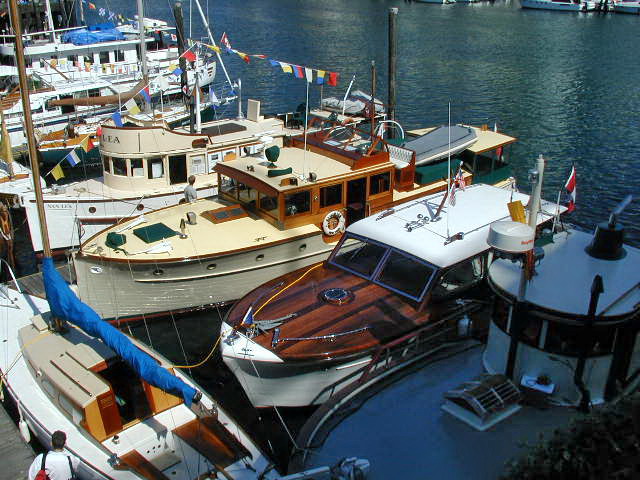In this detailed portrait image, we're looking down at a busy marina where a row of boats is docked, each flaunting unique designs and color schemes. The nearest boat, dark blue and shrouded in shadow, contrasts strikingly with the next, which features a wood and white mottled appearance, basking more in sunlight. Following this is a boat with rich brown wood tones, occupied by a man standing on it, facing away from us. Further along, we can see a beige boat with the partial name "Lea" visible at the top, and beyond this, several more indistinct vessels fading into the distance. The marina is adorned with colorful banners hanging from poles, adding a festive atmosphere to the scene. In the foreground, the edge of a pier is visible, with a person in a white t-shirt standing at the bottom left corner, also facing away from us. Another noteworthy detail is a small boat positioned horizontally near the pier, featuring a curled blue folded sail. Overall, this vivid scene captures about ten boats, set against the backdrop of water tinted with greenish aqua hues, embodying the tranquil yet lively spirit of the marina.